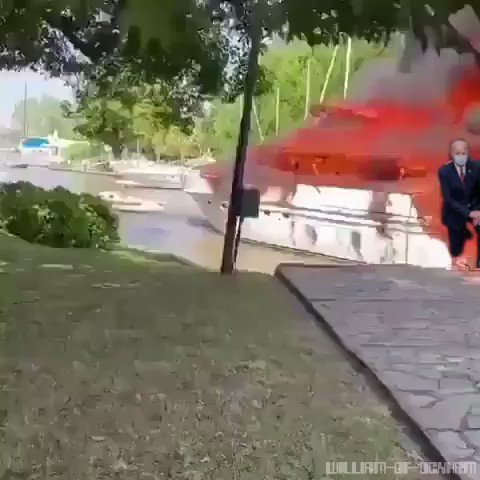The image is a square photograph depicting a river scene from the shore, featuring a mixture of natural and doctored elements. In the foreground, there is a grass-covered riverbank leading to a stone sidewalk. Centered prominently within the river is a large white boat, with its top section unnaturally colored in a striking red, accompanied by exaggerated gray smoke, giving the illusion of flames consuming the boat—an effect that appears clearly photoshopped. To the right of the boat, partially cut off and appearing superimposed, is a masked, suit-clad figure resembling President Joe Biden, sporting a red tie. This figure seems inappropriately placed, hinting at manipulation of the image. Surrounding the main subjects, the background features a lush display of vibrant green trees and additional boats dotting the river, adding a layer of natural scenery to the otherwise altered photograph.